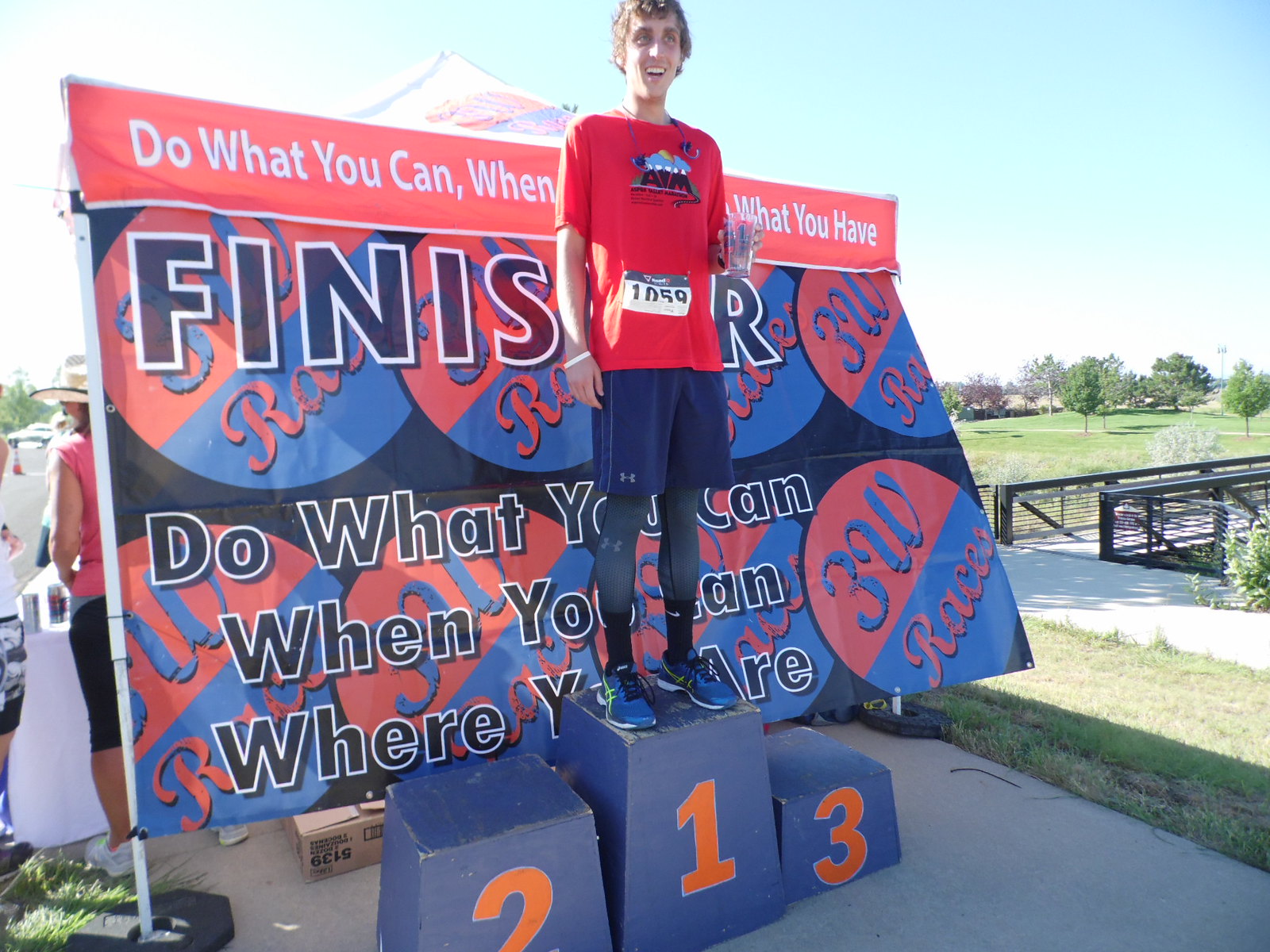In this outdoor photograph, a man is jubilantly standing on the first place podium of a three-tiered podium set, which is typically used for race winners. The podium, colored blue, has the numbers 1, 2, and 3; he stands on the highest tier marked with number 1. Dressed in a red t-shirt, blue shorts, gray compression pants, and blue running shoes, he is holding a glass-like object in his hand. Behind him, a large banner reads "Finisher" and contains motivational text such as “Do what you can, when you can, where you are,” although some words are obscured by his body. Further behind the banner, a grassy field with scattered trees and a small bridge on the right provide a picturesque backdrop against the clear blue sky. There's also a sidewalk where some people, possibly race organizers, are seen standing near some boxes, potentially filled with refreshments for the race participants. The overall scene indicates a celebratory moment after a race, epitomizing triumph and joy.